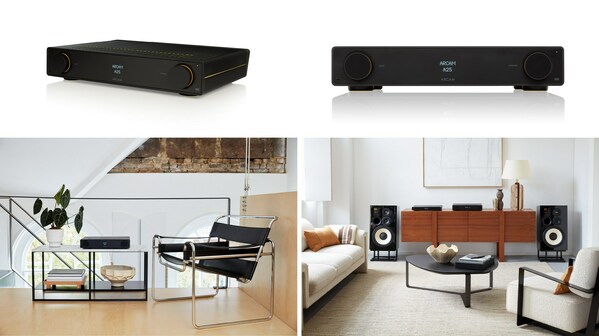The image is a collage of four pictures displaying a black rectangular electronic device, likely an amplifier, from different angles and settings. The top two pictures show this device against a solid white background. The left image displays it at an angle, revealing both the front and side, with knobs on either side, while the right image shows the front view. Both images depict a simple black rectangular amplifier with various control knobs and a screen with text.

Below these, the bottom left picture features a small modern living room scene with a glass table. On the table sits the same amplifier, accompanied by a potted plant and books. The room is furnished with a stylish black chair with wire-like arms and a thin back strap, suggesting a contemporary design. 

The bottom right picture reveals a more spacious living room setup. Here, the amplifier is placed on a long brown cabinet, beside what appears to be a smaller VCR-like device. The cabinet also houses two large speakers at either end, with a lamp sitting atop it. The furniture includes a white rocking chair on the right, a white sofa on the left, a brown coffee table with a vase and books, and a painting on the back wall, conveying a cozy and eclectic atmosphere.